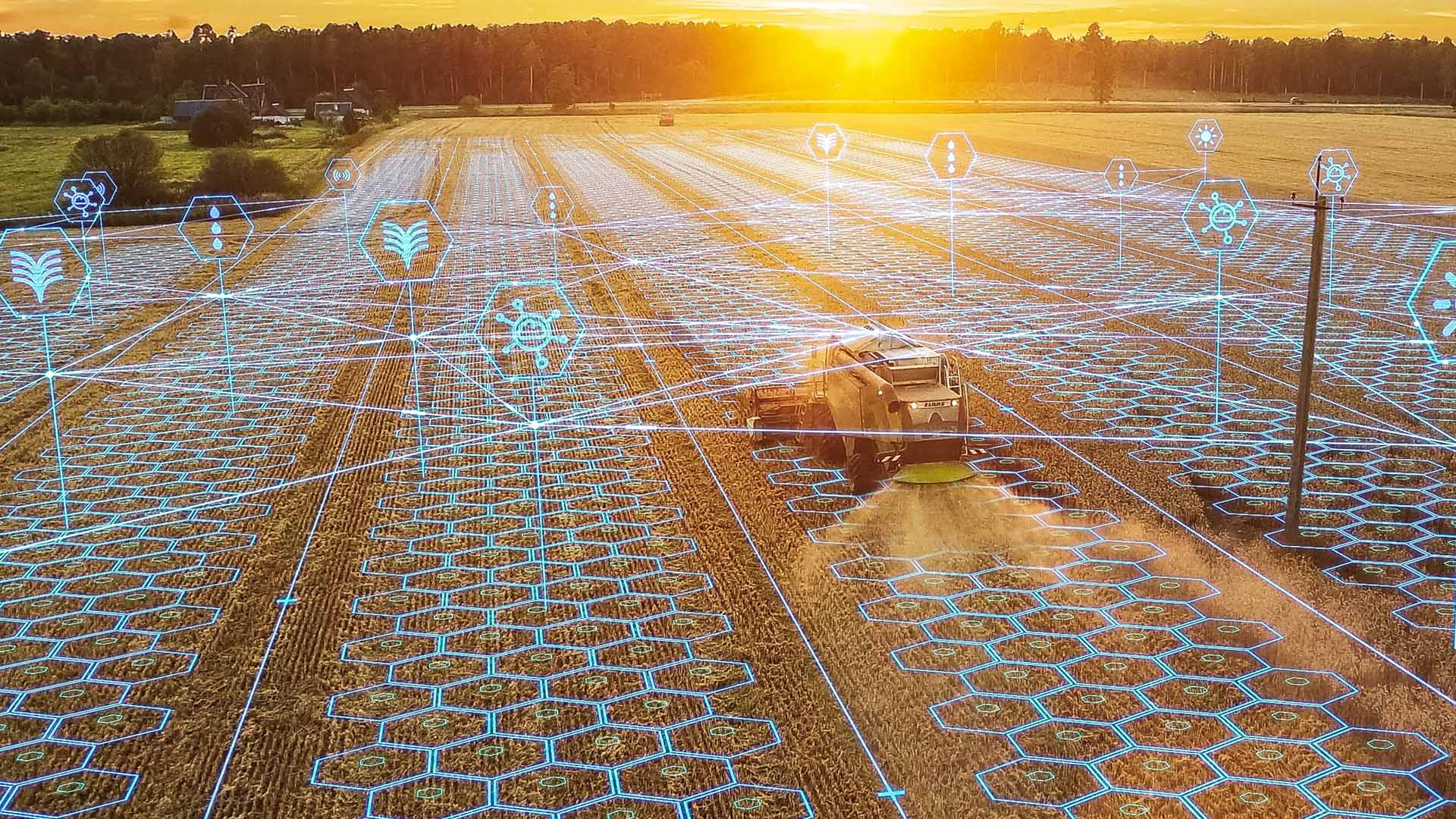An aerial view captures a vast farmland at either sunrise or sunset, bathing the scene in a warm, yellowish hue. In the foreground, a large tractor is prominently featured, making its way across the field, spraying a substance. The tractor is towing machinery behind it, emphasizing its agricultural role. The field, predominantly filled with crops, is overlaid with a translucent, blue hexagonal grid. This grid forms a network of interconnected hexagons, each marked with distinct icons such as viruses, wings, and dots, suggesting various conditions or monitoring points within the field. In the upper portion of the image, a grassy area and a line of trees can be seen, silhouetted against the setting sun. Distant buildings and a scattering of trees complete the tranquil yet technologically enhanced rural landscape.